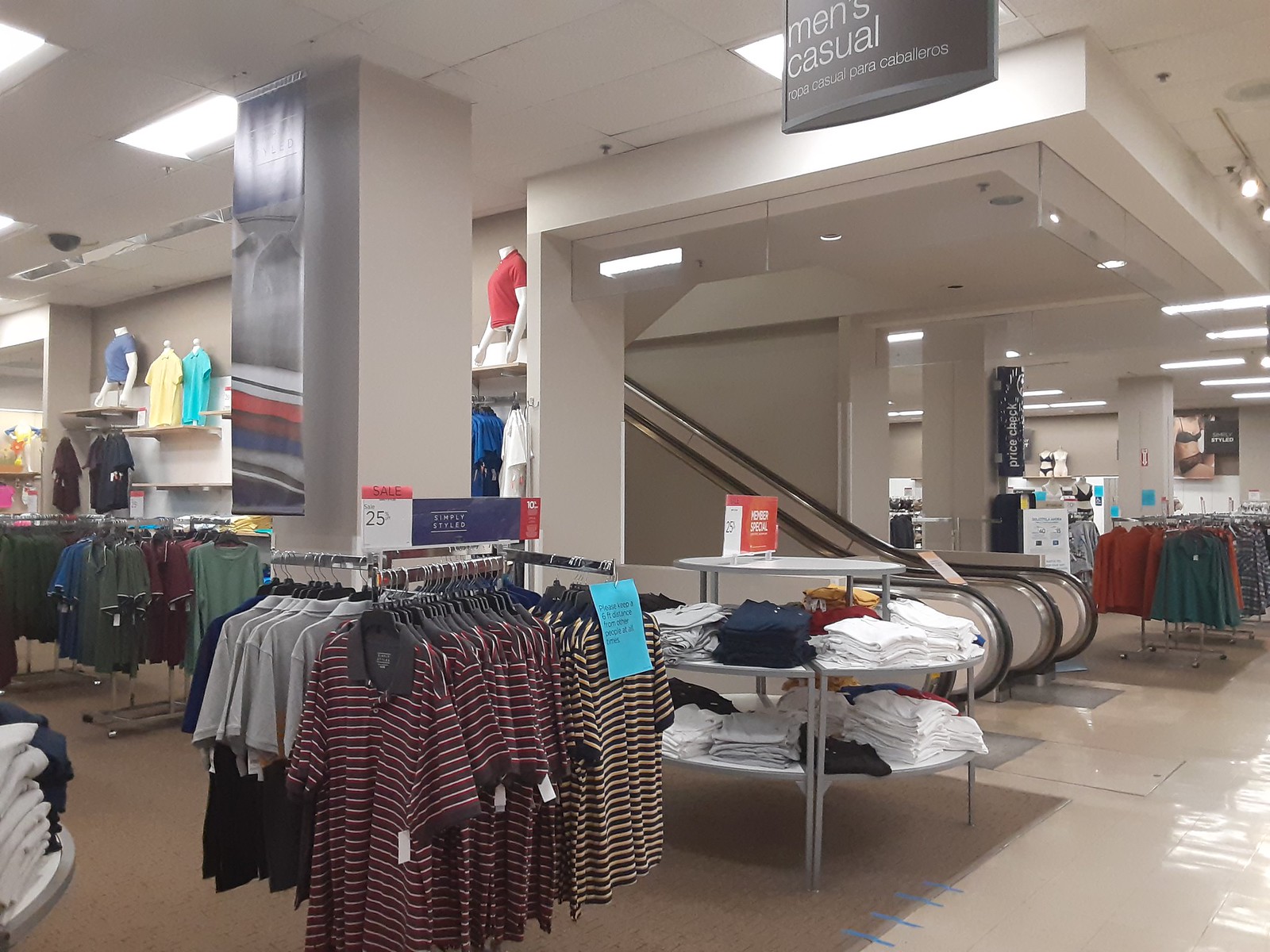This horizontal photograph, likely taken inside a department store reminiscent of Nordstrom, illustrates the men’s casual section prominently. The image captures a variety of striped polo shirts in shades including red, yellow, and black, some neatly folded on tables, others hung on racks against a light brown carpet. Noteworthy is a sign urging customers to maintain a six-foot distance. The backdrop reveals a shiny laminate floor extending towards black and silver escalators, framed subtly by fluorescent lights overhead, enhancing the store's well-organized ambiance.